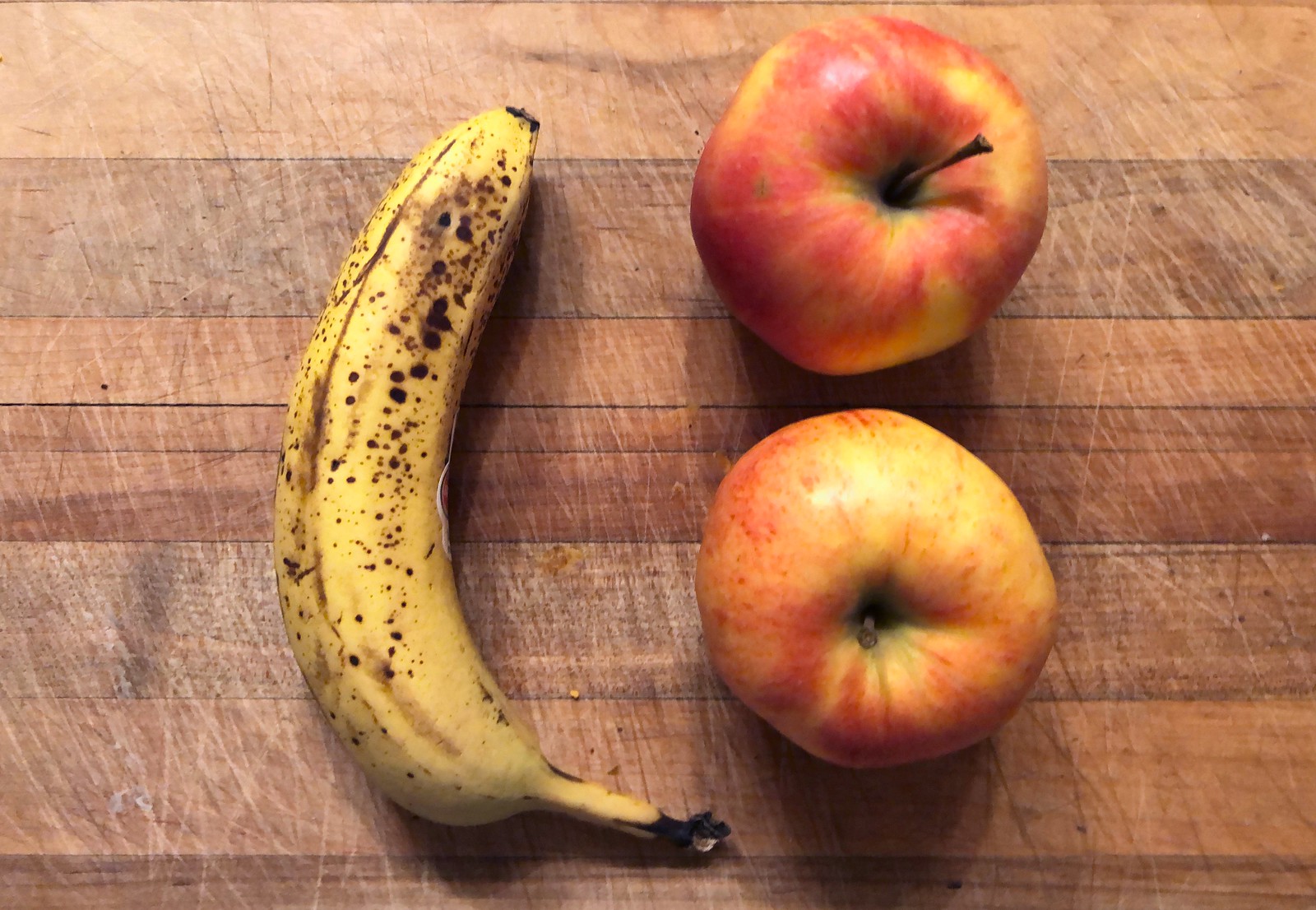An overhead shot captures a rustic wooden table, potentially doubling as a well-worn cutting board, adorned with a few nicks and marks that tell tales of past culinary adventures. On the left side of the frame rests a slightly overripe banana, its peel peppered with black spots and still bearing a sticker. Adjacent to the banana are two vibrant apples, their red skins shimmering with hints of yellow, and each one nudging the other like affectionate companions. The arrangement playfully resembles a smiling face, with the banana forming a cheerful smile and the apples representing bright eyes. Bathed in even lighting, this simple yet charming composition features just three pieces of fruit, invoking a sense of whimsy and freshness.